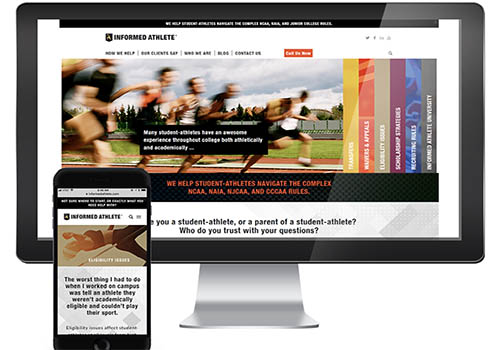This image features a computer monitor displayed prominently, anchored by a sleek silver base. On the monitor's left-hand side, a vertically-held cell phone screen is visible. At a magnification of 200%, the text on the phone is somewhat blurred and difficult to read but includes the heading "Informed Athlete." Beneath this title, legible text reads, "Are you a student athlete or a parent of a student athlete? Who do you trust with your questions?" 

A central, large photograph occupies a significant portion of the display, depicting a group of five or six runners in motion, their figures blurred to suggest movement. To the right of this photograph are six vertical rows in a sequence of colors: yellow, red, gray, purple, blue, and a deeper shade of gray.

Furthermore, the cell phone screen on the left side of the image showcases a horizontally-oriented picture of a female, accompanied by the label "Informed Athlete." Below her image, partially obscured text reads, "The worst thing I had to do when I worked out on campus was," followed by text that is not legible.